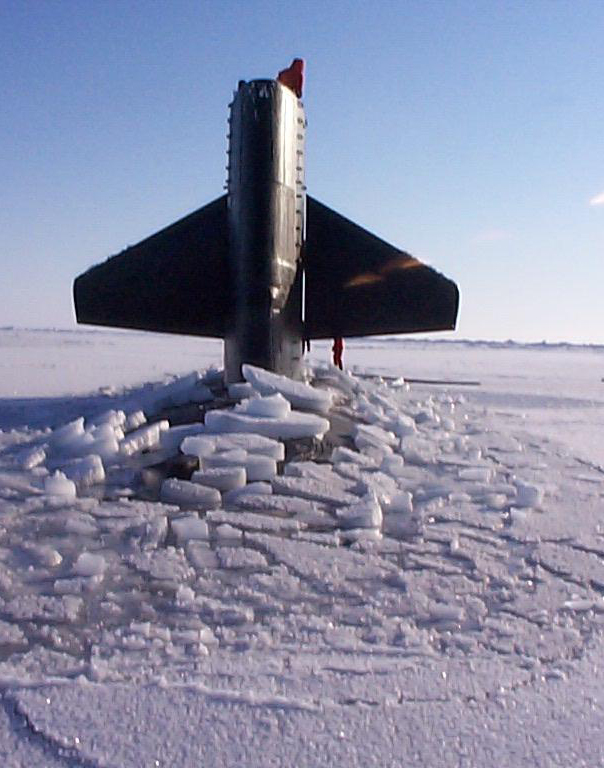In the photograph, a large metallic object—potentially the broken-off tail section of an airplane or submerged part of a submarine—pierces through a vast, ice-covered landscape. The scene is set amid a sprawling sheet of ice that extends to the horizon. This object, partially embedded and surrounded by jagged, shattered ice, stands angled into the frozen surface, indicating a dramatic impact or surfacing event. The object features chrome and brown elements at its base, with black wings or fins on either side, and is capped with a small red component. At the rear of this object, a lone figure, possibly a sailor or survivor, stands at a considerable distance, highlighting the expansive and isolated environment. Above this stark, icy terrain, the sky is a clear blue, growing lighter towards the bottom right, emphasizing the cold, bright atmosphere of the daytime setting.